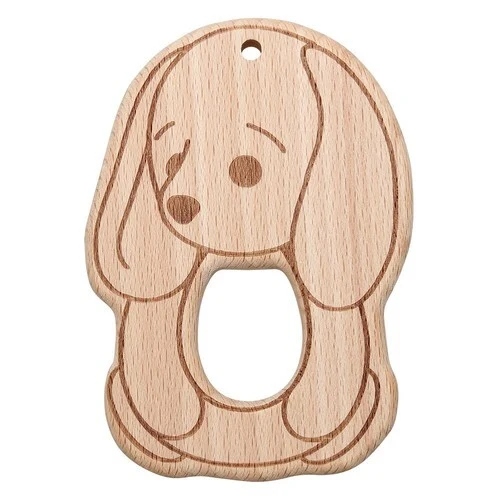This is a detailed wooden artwork featuring an intricately etched image of a sad-looking puppy. The entire object is crafted from light brown wood, showcasing visible vertical striations. The image on the wood, which might have been created through wood burning or painting, displays the puppy's face with large floppy ears, eyebrows, a brown strawberry-shaped nose, and a subtle hint of one eye, enclosed within an oval-shaped head. 

Below the head, there is a significant, almost egg-shaped cutout that mirrors an oval with its top part removed, positioned right underneath what would be the puppy's jawline. This hole runs completely through the object, giving it a resemblance to a large opening similar to a toilet seat.

The wood cutout includes additional artistic elements indicating the puppy's body and legs, which are depicted as simple, curved shapes and lines. The primary body section below the head looks closer to a rounded egg shape, while the legs beneath are fashioned like elongated hot dogs with curves at the top.

The top of the object has a small, purposefully drilled round hole, allowing it to be easily hung for display. The design is enriched with the darker and lighter shades of brown, adding depth to the puppy's depiction. The artwork's shape gently curves with indented sides, giving it a smooth and elegant profile that could potentially serve as a functional yet decorative piece, such as a uniquely shaped cutting board or a hanger for lightweight items. This beautiful piece stands out as an artistic and possibly utilitarian wooden object.